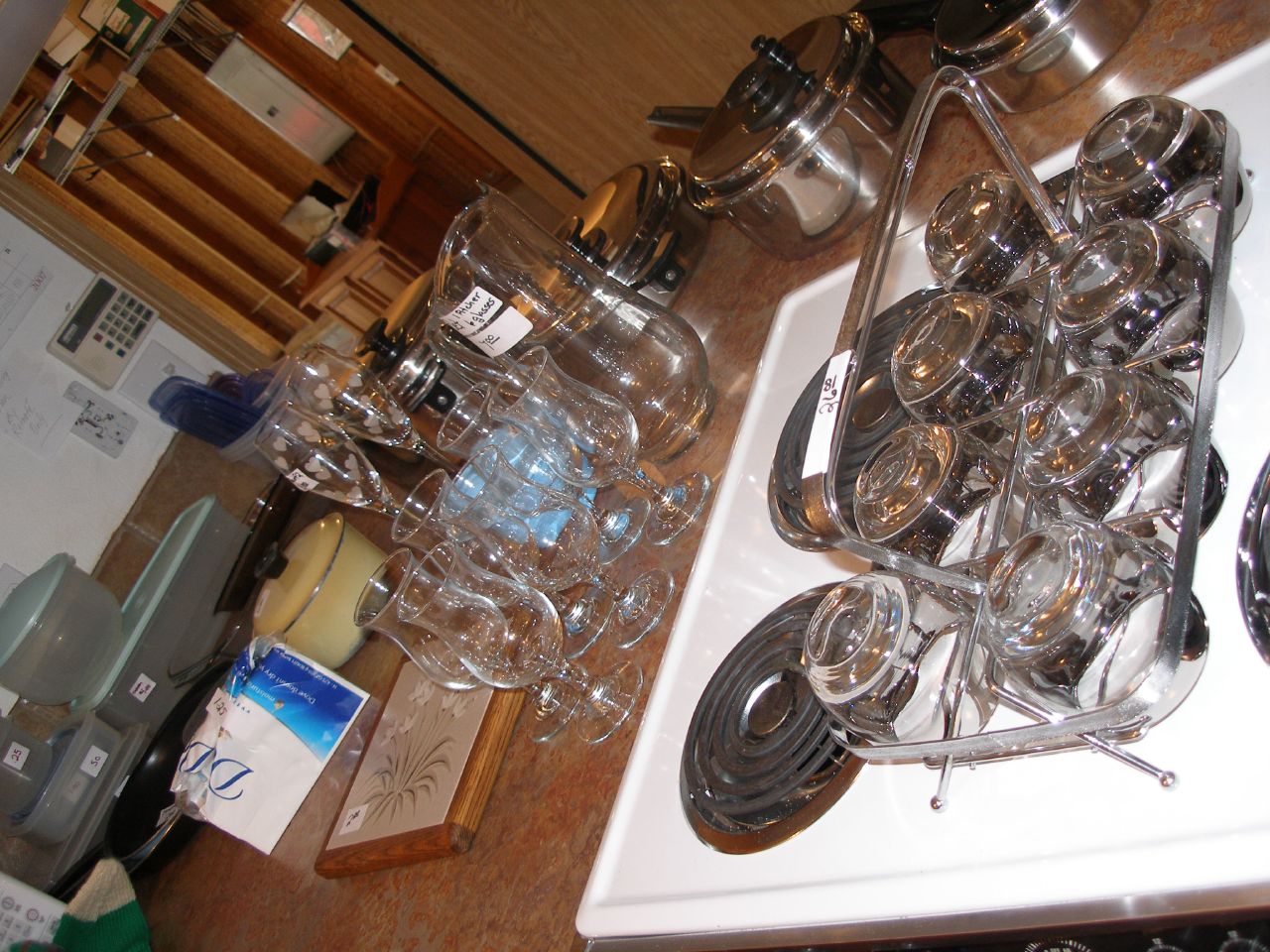The image showcases a bustling kitchen counter. On the right side, a white stove with black burners holds a large, silver tray bearing eight short, clear drinking glasses, neatly arranged for easy carrying. In the foreground, aligned on the countertop, several stainless steel pans gleam under the light. To the left, near the sink, a collection of whiskey snifters, characterized by their short stems and bulbous shapes, are accompanied by a tall glass pitcher. The countertop itself is dark and appears to be made of a durable plastic-like vinyl. One notable clutter is a ripped package of Dove soap lying in the midst of the items. Scattered among the repasts are a few elegant wine flutes. From the vantage point of the image, the background reveals another room, possibly an office or garage, marked by unfinished walls and a visible power panel in the upper-right corner, hinting at ongoing renovation or multi-functional space usage.